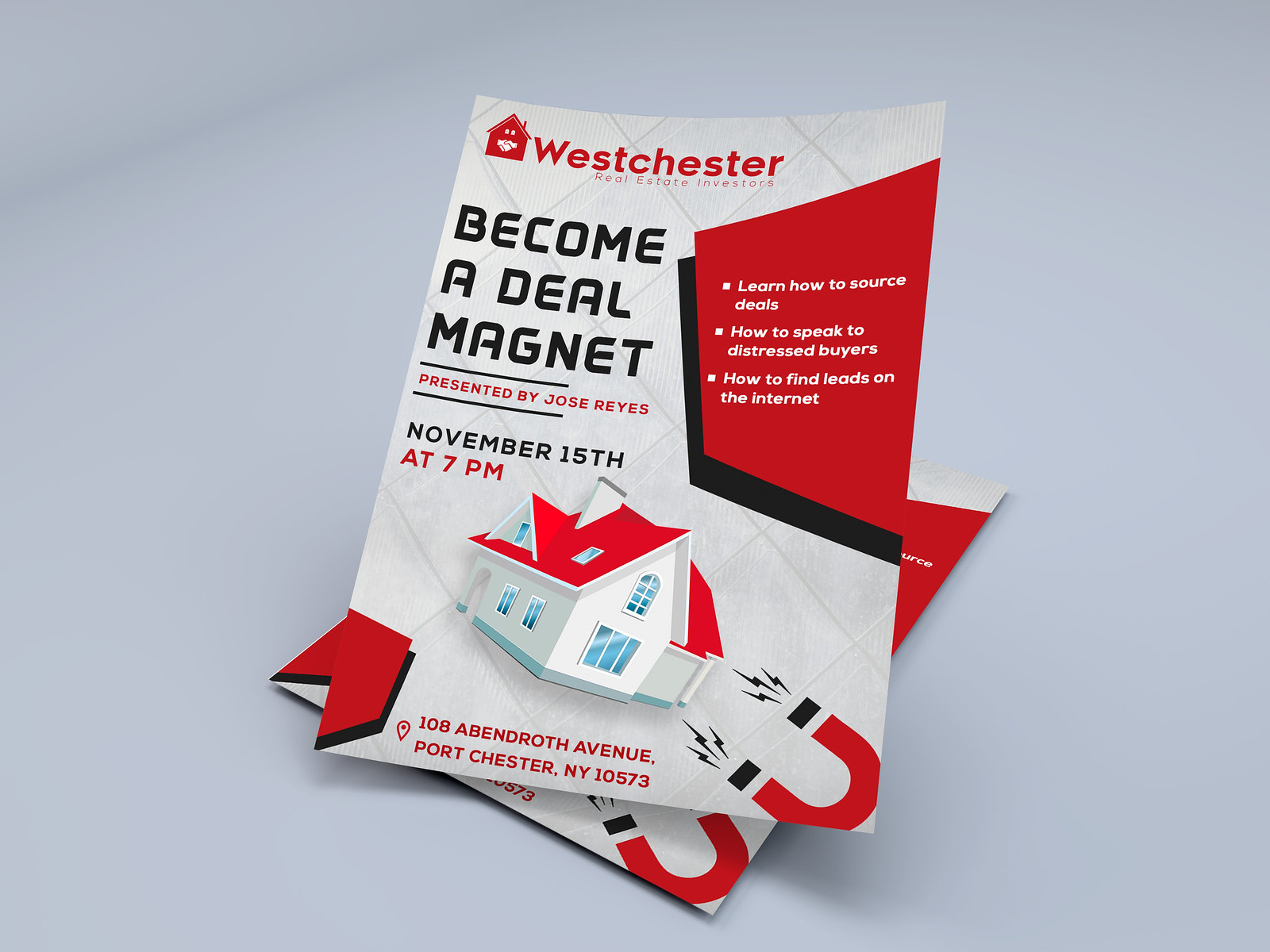The image features a large, square digital rendering of a promotional poster with a medium gray, tiled background. At the center of this background, there is a tall, rectangular brochure that seems to be floating slightly, tilted to the right, above a flat stack of identical brochures. The visible brochure is predominantly white with red and black text. 

At the top left corner, there's a small red illustration of a house with the text "Westchester" in red letters next to it, followed by "Real Estate Investors" in smaller red font. A large, bold, black text, left-aligned, reads "BECOME A DEAL MAGNET." Below, a horizontal black line separates this from the red text, "Presented by Jose Reyes," which is also bordered by black horizontal lines above and below it. The date "November 15th" is printed in black, followed by "at 7 PM" in red.

Near the bottom, a white house with a red roof and blue windows is depicted. To the lower right of the house, a red horseshoe magnet with black lightning strike symbols is illustrated, symbolizing the concept of attracting deals. The bottom of the brochure additionally includes an address: "108 Abendroth Avenue, Port Chester, New York, 10573."